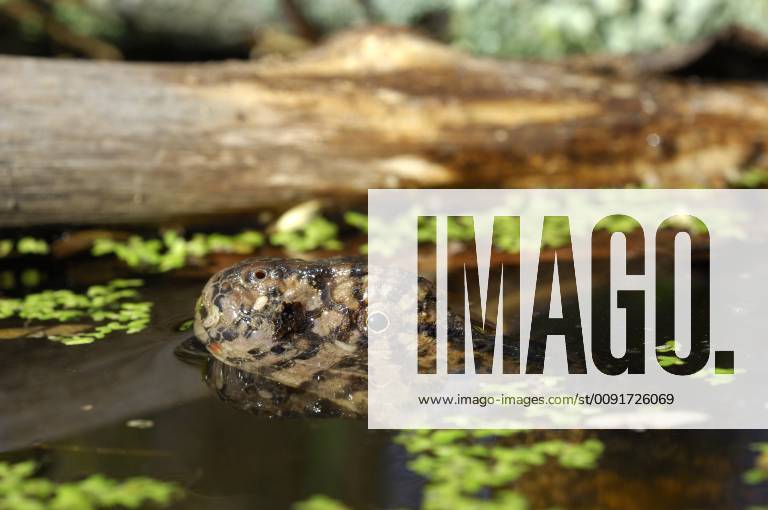This close-up outdoor color photograph captures a reptilian head, likely a lizard or snake, partially submerged in a pond of murky, dark brown to black water fringed with tiny green floating plants. The reptile's eye and nostril are visible, protruding above the water's surface. Its skin displays a mottled pattern of black and brown, with some tan stripes. Dominating the lower right quadrant of the image is a heavily watermarked logo that reads "IMAGO." Beneath this, a barely visible web address, www.imago-images.com/eskimo/0091726069, further obscures the details. In the background, a horizontally positioned log, slightly rotted and blurred, stretches from the left to the right, providing a natural, out-of-focus backdrop to the sharply detailed foreground.